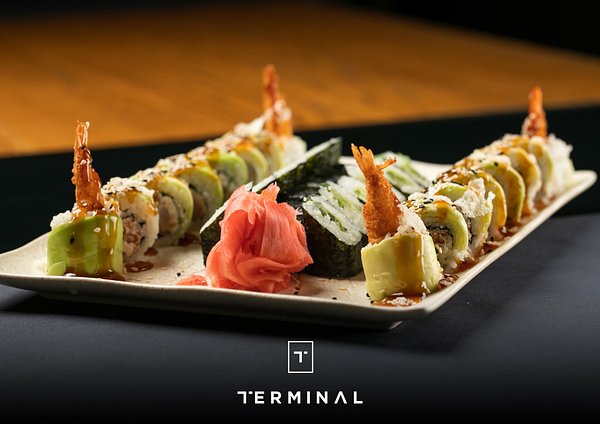In this professionally shot photo, presented as a display for the restaurant "Terminal," a rectangular white glass serving tray is diagonally oriented on a black cloth with a minimalist logo featuring a T in blocky white lettering. The tray holds three meticulously arranged rows of sushi, set against the blurred backdrop of a wood table.

The first and third rows feature sushi rolls enveloped in light green avocado slices, draped over white rice with a brown and black filling, punctuated by crispy golden fried shrimp tails rising from their centers. The middle row consists of sushi wrapped in black seaweed, filled with white rice and green vegetables, and accentuated by a bright coral pink piece of ginger. An orange-brown sauce, potentially spicy or a duck fish sauce, artfully drips around the sushi, enhancing the dish's vibrant color palette that ranges from white and pink to green and black.

This exquisite composition highlights the diversity and artistry of sushi, capturing both its visual appeal and culinary craftsmanship.